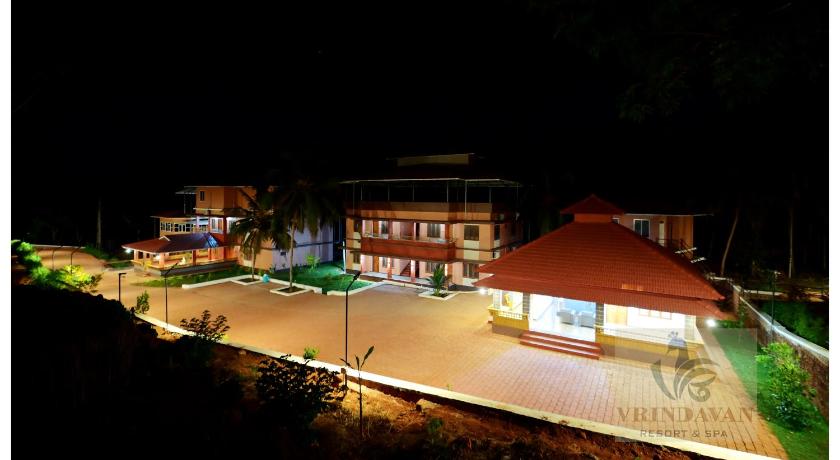This vibrant nighttime photograph captures the stunning exterior of the Vrindavan Resort and Spa. Positioned on a hill, the view encompasses three multi-story buildings with prominent brick facades and brown-orange hues. The well-lit structures are accentuated by a red-tiled stucco roof, particularly noticeable on what appears to be a pool house to the right. The expansive patio stretches across the front of all three buildings, framed by meticulously manicured grass areas and a variety of trees, including striking palm trees. The sky is dark, reinforcing the nighttime setting, while strategically placed lighting bathes the property in a warm, inviting glow. In the bottom right corner, a faintly visible silhouette of a peacock serves as the resort's logo, accompanied by the text "Vrindavan Resort and Spa," subtly integrated into the image.